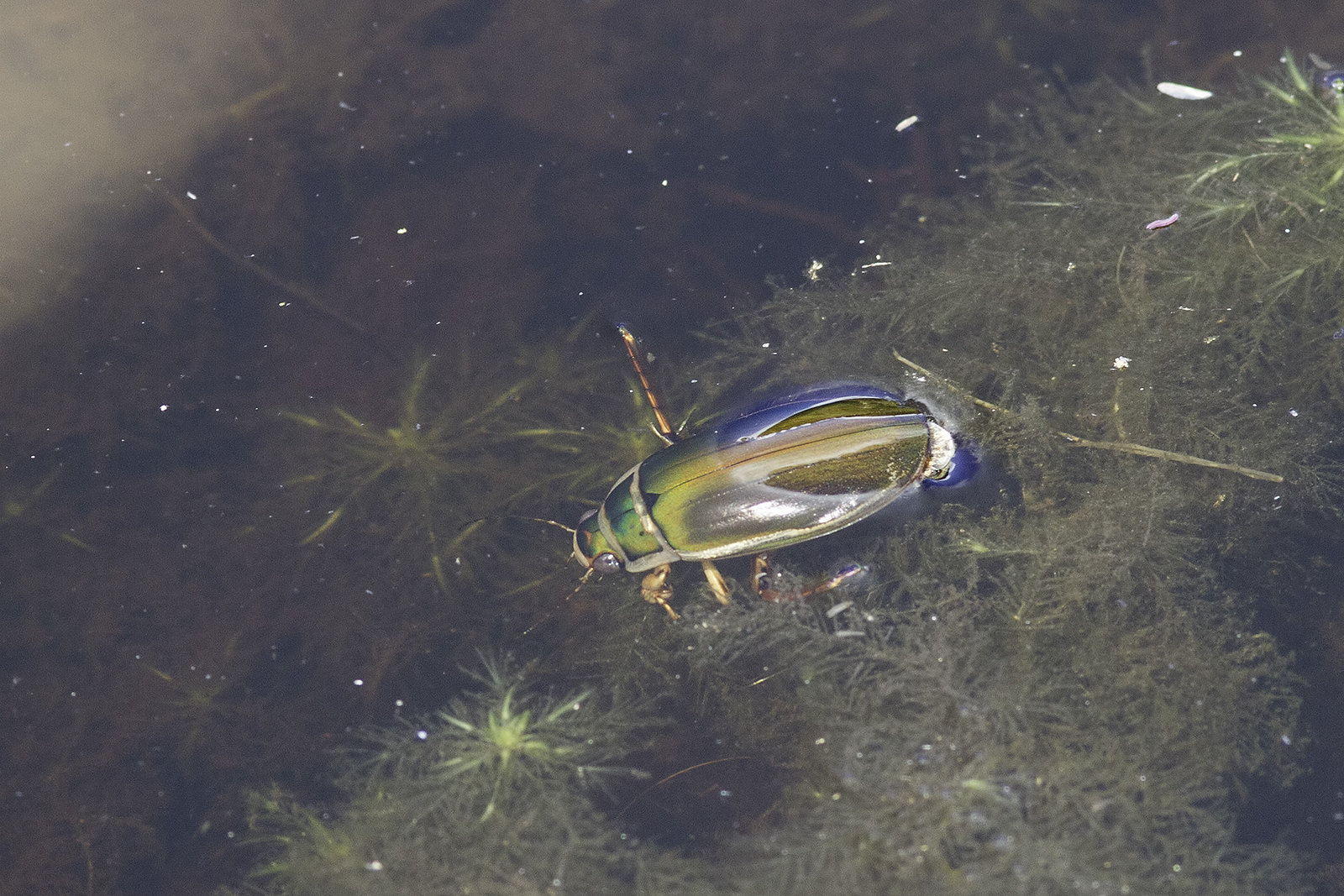A high-quality, brightly-lit daytime photograph showcases a solitary water beetle partially submerged, with half of its body rising above the water's surface. The beetle's fine details and the surrounding environment are captured in vivid color. Lush green grass fringes the water, providing a natural backdrop to the scene. The clarity of the image highlights the serene and undisturbed setting, emphasizing the beetle as the sole focal point with no other insects, people, or vehicles present.